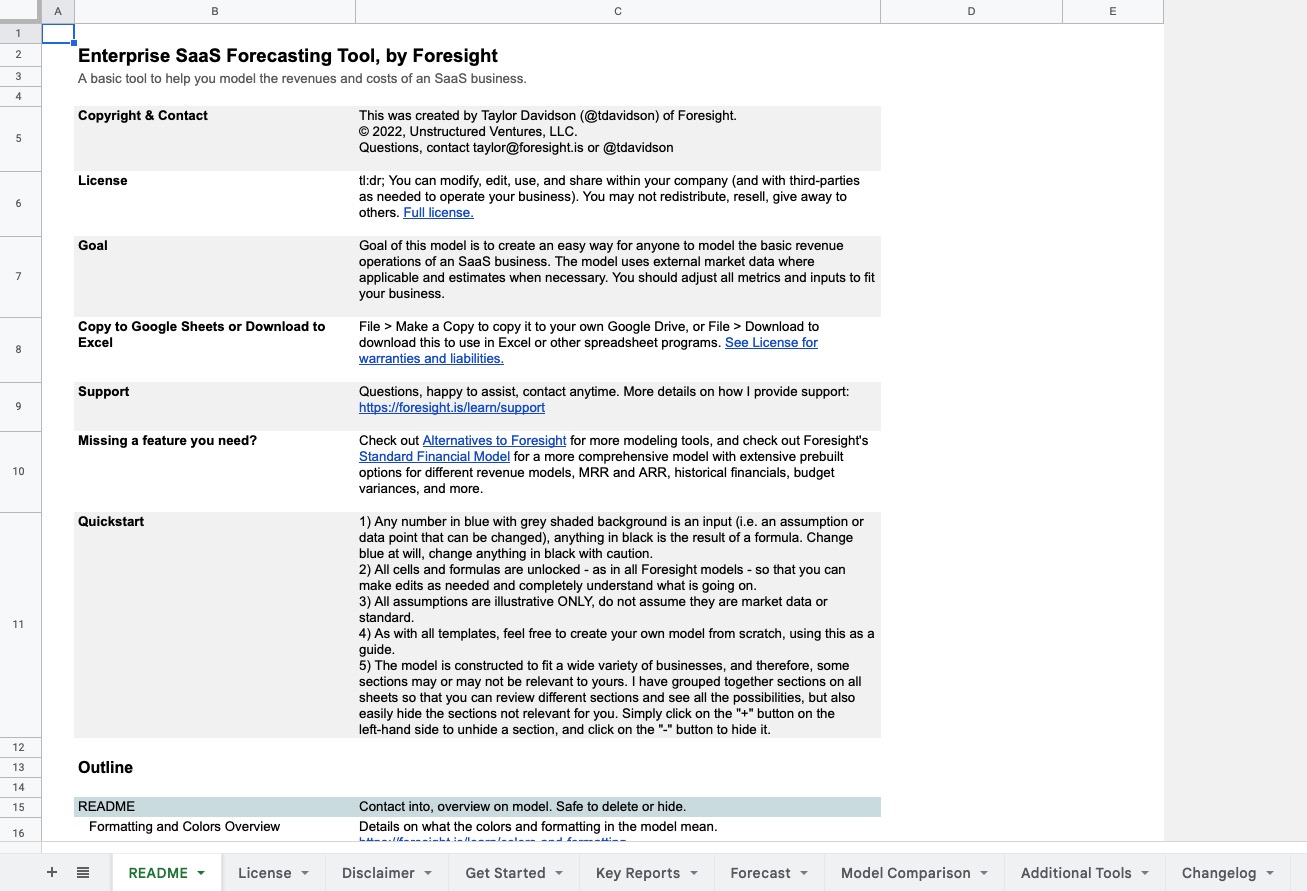**Caption:**

A detailed screenshot of a forecasting tool template designed in a familiar spreadsheet format, such as Excel or Google Sheets. At the top, recognizable column headers labeled ABC are visible alongside row numbers 1 through 16 on the left. The main content area has a pristine white background, and prominently featured is the title: "Enterprise SaaS Forecasting Tool, by Foresight," written in clear, capitalized and lowercase letters. Beneath the title, in smaller, gray font, a subtitle describes the tool: "A basic tool to help you model the revenues and costs of a SaaS business."

The template is divided into alternating sections with light gray and white backgrounds. The first light gray section, in small, bold black lettering, is labeled "Copyright and Contact." To the right, in non-bold text, is a credit note: "This was created by Taylor Davidson (at T. Davidson of Foresight). Copyright 2022 Unstructured Ventures, LLC. Questions, contact Taylor at foresight.is or at T. Davidson."

Following this, a white background section features the heading "License" in bold black font. Beneath, in regular font, it succinctly states: "TL;DR: You can modify, edit, use, and share within your company (and with third parties as needed to operate your business). You may not redistribute, resell, give away to others." An underlined, blue clickable text labeled "full license" invites users to access more detailed licensing information.

Another light gray section follows, titled "Goal" in bold text. To the right, non-bold text elaborates: "The goal of this model is to create an easy way for anyone to model the basic revenue operations of a SaaS business. This model uses external market data where applicable and estimates when necessary. You should adjust all metrics and inputs to fit your business."